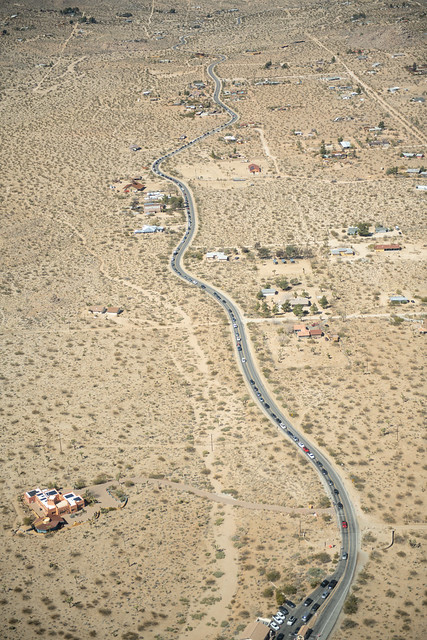This aerial photograph captures a winding gray asphalt road cutting through a barren, desert-like landscape. The road, bustling with vehicles and displaying heavy traffic, spans the entire vertical axis from top to bottom. Surrounding this main roadway is a vast expanse of sandy terrain dotted with several grayish-green bushes and cacti. Sparse patches of dull, greenish plant life contrast against the predominant brown earth. Numerous dirt roads branch off from the main highway, leading to scattered adobe-style buildings and residential houses, which are few and far between in this rural area. Notably, the foreground to the left showcases a more elaborate structure, potentially a gazebo, adding a hint of architectural variety to the scene. As the image extends into the distance, the density of visible structures decreases, although a few industrial-looking complexes and residential communities are discernible, giving way to the expansive desert that dominates the photograph.